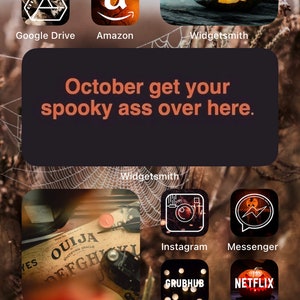The screenshot displays a Halloween-themed mobile phone interface adorned with intricate spider webs over a brown and gray background. The wallpaper features eerie elements, possibly including spiders and bones. Prominently showcased at the top are icons for Google Drive, Amazon, and Widgetsmith. The lower left corner is highlighted by a Ouija board icon, followed by distinctly styled app icons for Instagram, Grubhub, Messenger, and Netflix, all exhibiting Halloween motifs. A significant feature in the center is an oversized widget, spanning four icon spaces in width and two in height. This dark brown widget, with vibrant orange text, reads, "October, get your spooky ass over here," and is labeled underneath with "Widgetsmith." The use of Widgetsmith allows the customization of the phone's interface, seamlessly tying the icons and overall color scheme into a cohesive Halloween theme. Notably, the Netflix icon has been transformed to include a jack-o’-lantern, exemplifying the themed customization applied throughout the interface.